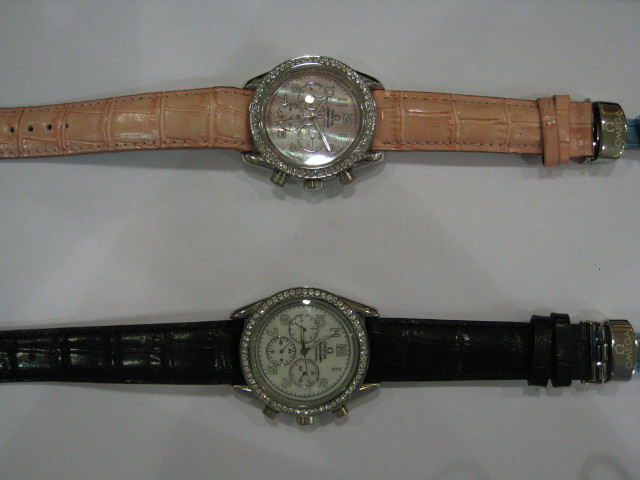On a pristine white background, two exquisite watches are displayed, one above the other. The top watch features a chic pink leather band, embossed with an elegant crocodile or alligator skin pattern. This band is secured with two small leather straps and a polished metal clasp. The watch face, encircled by a ring of glistening diamonds, showcases a classic clock layout with numbers 1 through 12 arranged clockwise. Additionally, the face is enhanced with three smaller sub-dials, meticulously placed, along with distinctive minute and hour hands.

Beneath it lies a striking watch with a luxurious black leather band, also styled in a crocodile or alligator skin pattern, mirroring the sophistication of the pink one. The black watch, branded with the prestigious name Omega, presents a similar numeral arrangement on its face, with numbers 1 to 12 displayed clockwise. Its dial is further adorned with three miniature clocks configured in a triangular formation, with two sub-dials positioned at the top and one at the bottom. Both timepieces exemplify refined craftsmanship and timeless elegance.